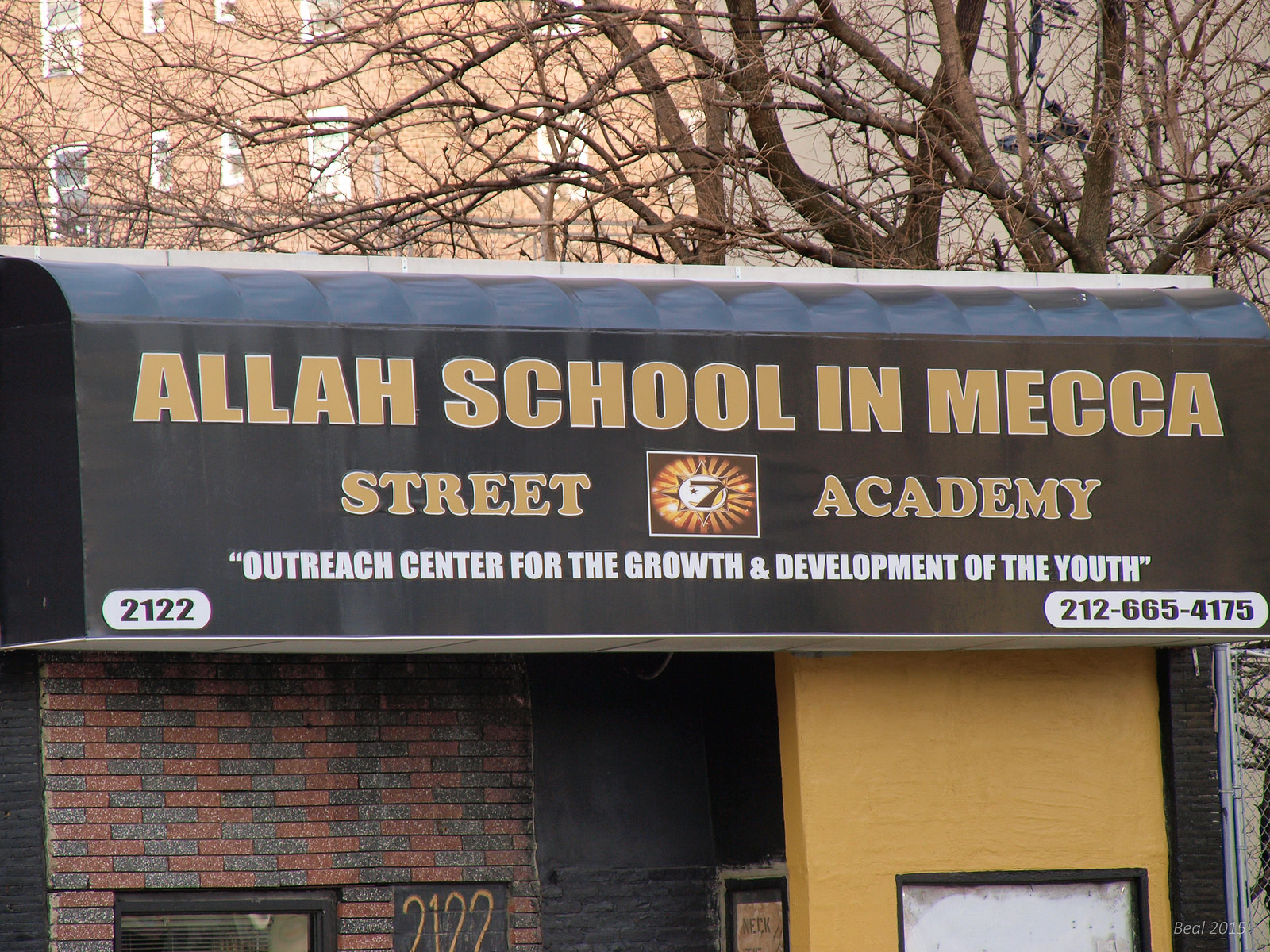The image depicts the front of a business building with a black awning prominently displaying gold and white text. The top of the awning reads, "Allah School in Mecca," followed by "Street Academy," with a logo of a sun and a number seven illuminated by golden lights in between. Beneath this, the text reads, "Outreach Center for the Growth and Development of the Youth." The bottom left corner of the awning shows the address "2122," while the bottom right corner lists a phone number, "212-665-4175."

The building itself features a façade with a distinctive mix of architectural styles: the left half is constructed with a combination of red and black bricks, and the right half is a smooth yellow stone. A window is visible on the lower left side of the building. To the right of the building, there is a chain-link fence.

In the background, there is a tall, motif-floored red brick building with two floors of visible windows on the left and a dark brown building without visible windows on the right. Towering above the building are several tree trunks with numerous branches but no leaves, indicating that the season might be either fall or early spring. The sky is visible in the upper right corner of the image.